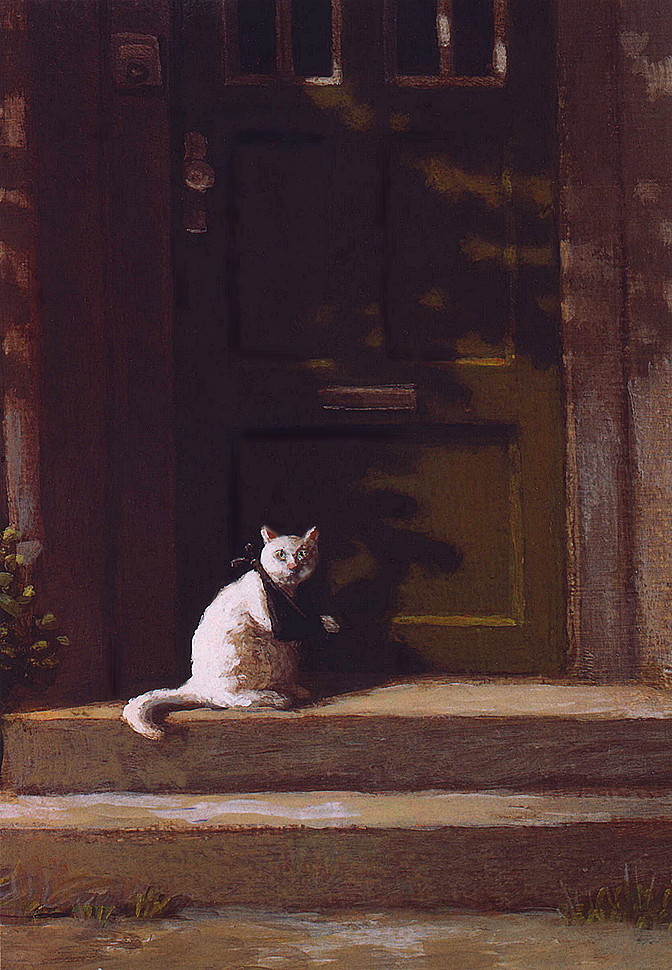The painting "The Broken Paw" by Michael Sowa is an evocative color oil painting in a portrait orientation, rendered in the style of Surrealism Animal Painting. It features a white cat sitting on the top of two light brown concrete or terracotta steps. The cat, gazing up at the viewer with bright turquoise green eyes, has a broken right paw encased in a black sling. Details like the cat's pink nose, the pink inside its ears, and its long curved tail hanging over onto the step add lifelike touches. Behind the cat is a brown wood door with a golden knob, a hinged mail slot, and a few visible panes at the top. Flanking the steps are small patches of grass and glimpses of a bush with yellow flower buds, hinting at the natural setting around this domestic scene.